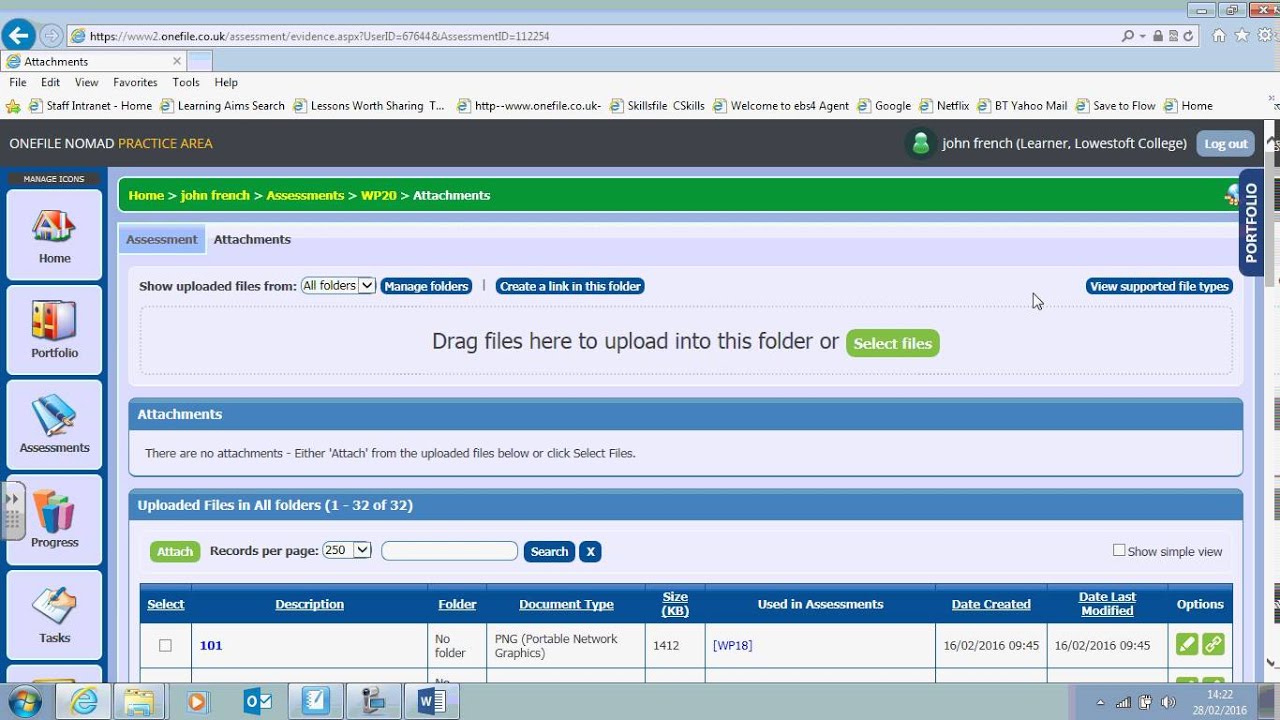The screenshot captures the view of a computer screen displaying a webpage, likely from the website "onefile.co.uk." At the top of the window, there is a search bar displaying the web address and an open tab navigated to the attachments section. Below the tab bar, the standard menu options are visible: File, Edit, View, Favorites, Tools, and Help.

The toolbar beneath offers various site navigation options labeled as Staff, Internet, Home, Learning, AIM Search, Lessons Worth Sharing, Skill File, Welcome To, eBoil, Agent, Google, Netflix, Yahoo Mail, Save to Flow, and Home.

The main content on the screen shows the "Onefile Nomad Practice Area." On the left, a sidebar contains options like Home, Portfolio, Assessments, Programs, and Tasks represented by square icons. At the top center of the main area, there is a section labeled "Drag files here to upload or select file" indicating an area to upload files. The central part of the screen is designated as the attachment section, and at the bottom, there is a list titled "Uploaded files in all folders" accompanied by a search bar.